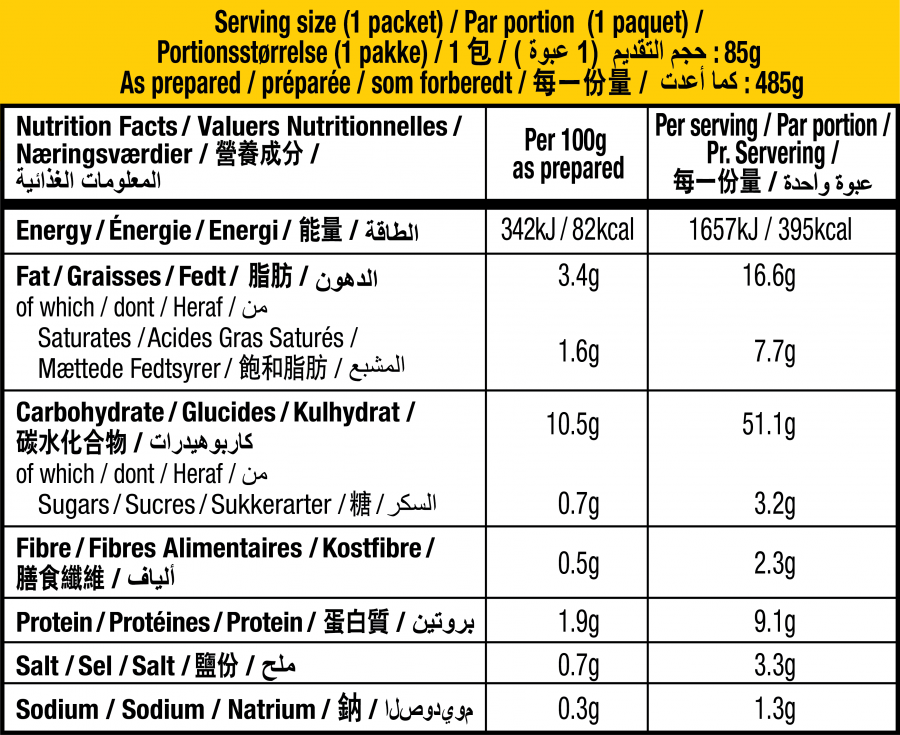The image depicts a Nutrition Facts label that is presented independently of any packaging. The label is a square shape with a distinctive gold band across the top. The background is gold, while the text is rendered in black. At the top, the label states "Serving Size: One Packet," followed by translations in several other languages. Below, the label notes "As Prepared," though the text is somewhat difficult to read due to the multilingual content. 

The main background of the label is white, and the text within this section is black. The header "Nutrition Facts" is prominently displayed, followed by a section that states "per 100 grams as prepared." To the right, there's a corresponding column labeled "per serving." 

The first nutrient listed is "Energy," which is also translated into approximately four other languages. The energy values are presented in two columns: the first indicating 342KJ / 82KCAL and the second showing 1657KJ / 395KCAL. 

Subsequent sections of the label list other nutritional components, each accompanied by translations. These include "Fat," "Carbohydrate," "Fiber," "Protein," "Salt," and lastly, "Sodium." The specific numerical values for these components are not detailed in the description provided.